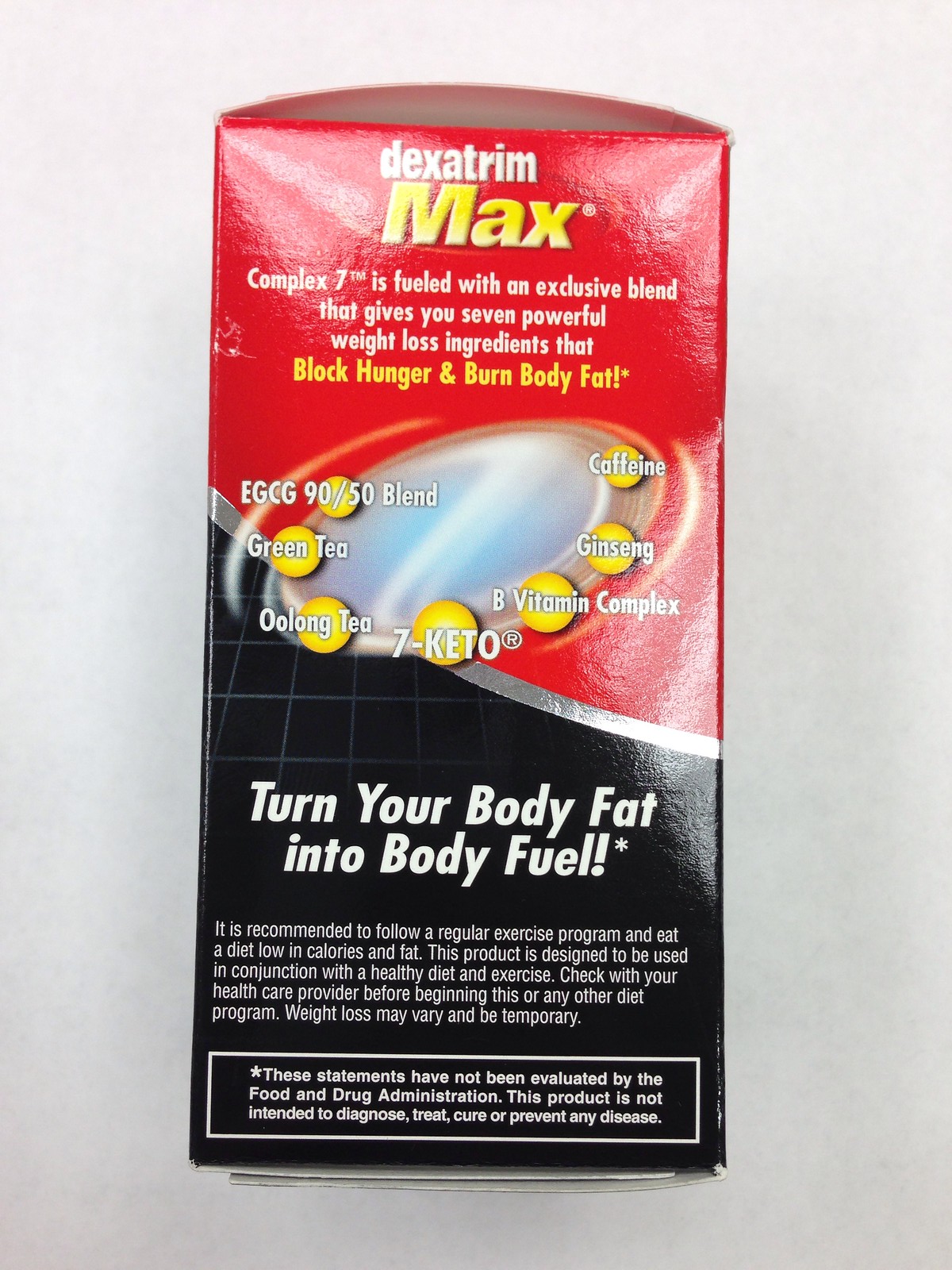This photograph captures a package of Dexatrim Max placed on a white or possibly gray table. The packaging itself features a striking color scheme: red at the top which transitions into black at the bottom, with a silver strip dividing the two sections horizontally. The package appears to be made of either plastic or paper and stands vertically.

At the top of the package, "Dexatrim" is prominently printed in white text. Directly below it, "Max" is displayed in bold yellow letters. Following this, in smaller white text, it states: "Complex 7 is fueled with an exclusive blend that gives you seven powerful weight loss ingredients." Highlighted in yellow against a white background, it claims to "block hunger and burn body fat." 

The bottom of the package encourages consumers with the phrase, "Turn your body fat into body fuel," written in white text.

Centrally located on the packaging, there's a U-shaped arrangement of seven small yellow circles, each labeled with a specific ingredient in white text, including caffeine, ginseng, and green tea. Additional regulatory and informational text appears in a white rectangular box at the bottom of the package, indicating, "These statements have not been evaluated."

Overall, the detailed design and color scheme of the Dexatrim Max packaging are intended to catch the eye and communicate its purported weight loss benefits.